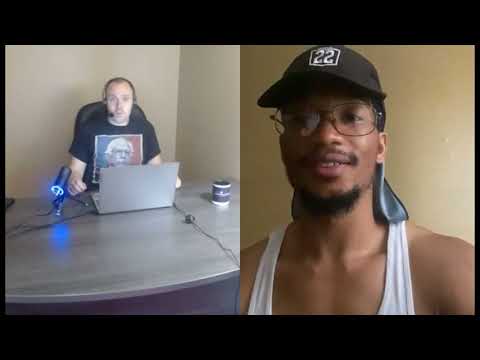This full-color, square image features two separate photographs within a single black-bordered frame. The borders on the top and bottom are thicker than those on the sides. The left side of the image shows a Caucasian man seated at a desk cluttered with various items, including a computer, coffee cup, and both a desk microphone and a headset microphone. He is wearing a black t-shirt emblazoned with an image of Bernie Sanders and is using a laptop with visible cords connected to it. His expression suggests focus, possibly engaging in a task such as gaming.

The right side of the image features a young African-American man standing against a beige wall. He sports a mustache, a chin beard, and black-framed glasses. On his head, he wears a black cap with the number '22' and what appears to be the tail end of a do-rag extending to protect his neck. His outfit consists of a sleeveless white t-shirt that highlights his well-defined shoulder muscles. He appears to be talking, with his mouth slightly open, showing the top row of his teeth. The overall composition of the photograph suggests a juxtaposition of two individuals engaged in different activities within their own separate environments.